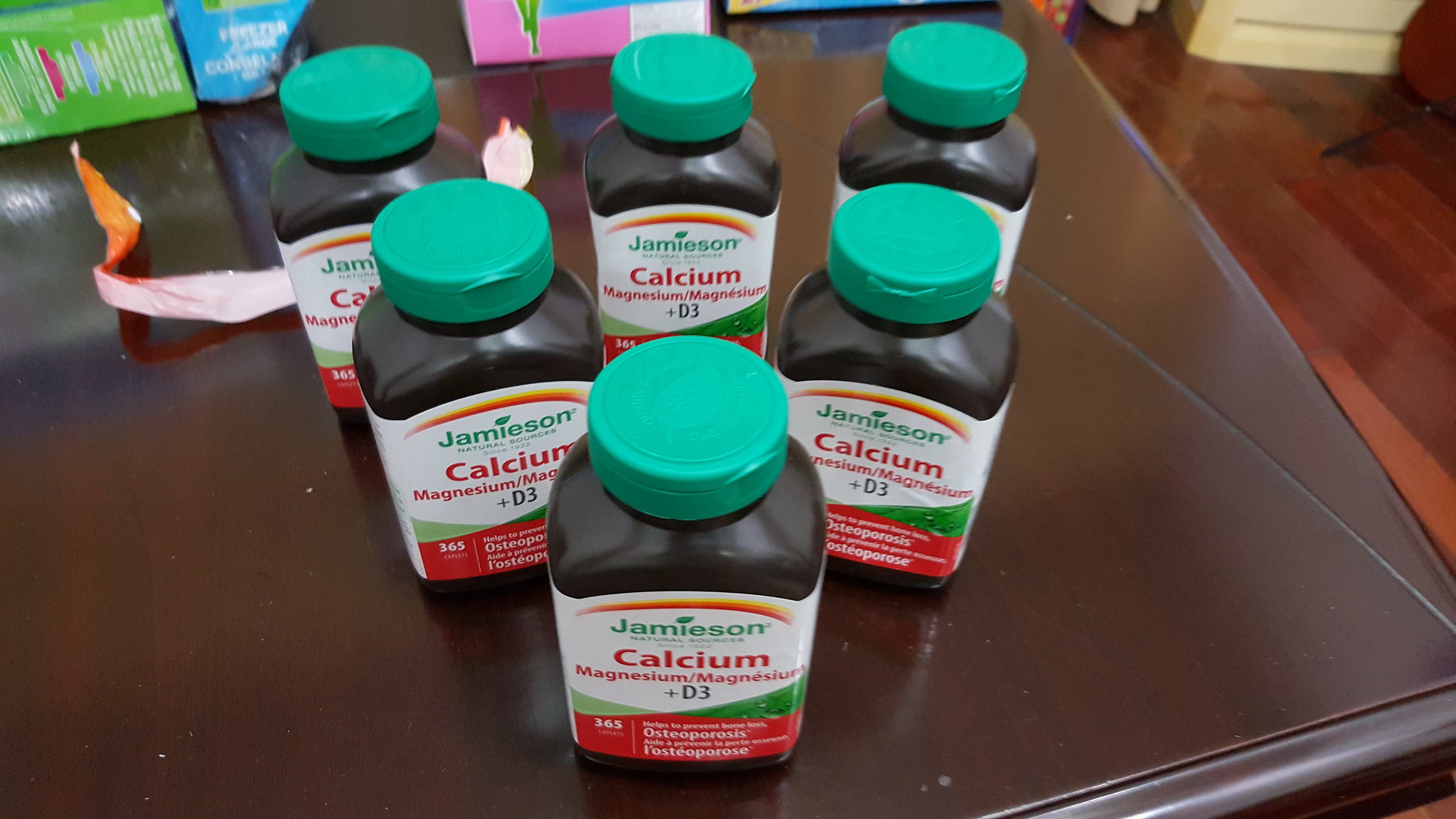The photograph captures a carefully arranged display of six dark plastic bottles of supplements, identified as calcium, magnesium, and D3, on a glistening, dark wooden table. Each bottle features a distinct green cap and a prominent white label. At the top of the label, the brand name "Jamieson" is spelled out in light green lettering with the letter 'I' stylized as a tree. Beneath this, there is an orange and yellow curve and some small, hard-to-read green text. In bold red letters, the word "CALCIUM" is visible, followed by "MAGNESIUM" with an accent over the 'E', suggesting a foreign spelling. The words "PLUS D-3" appear in dark bold lettering. At the label's bottom, a red section contains white text, with "365" on the left and references to osteoporosis on the right. The bottles are arranged in a triangular formation: one at the front, two directly behind it, and three more further back. The vibrant background details include a wood floor and colorful boxes that add context to the interior setting. The entire arrangement emphasizes the product's branding and claims, creating a visually informative composition.